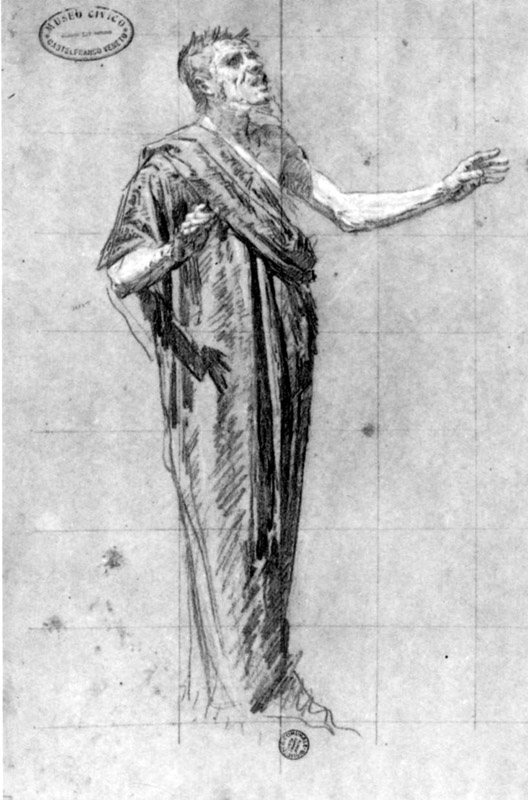The image is a detailed black-and-white drawing depicting a man, possibly a monk, saint, or preacher, in a long, flowing robe that drapes over his shoulder and extends down to his unseen feet. The man is positioned centrally, facing the top right of the image with a desperate and sad expression on his upturned face. He has short hair and appears to be extending both arms outwards towards the right, as if addressing or reaching out to someone. The background is comprised of a pattern of grey and white squares or rectangles, with subtle shading and splotches of grey, lending a realistic but not hyper-realistic quality to the artwork. Above the man's head in the upper left corner is a tiny, unreadable icon resembling an oval with printing in the center, presumed to be a trademark. A similar small black circle can be found beneath the drawing.